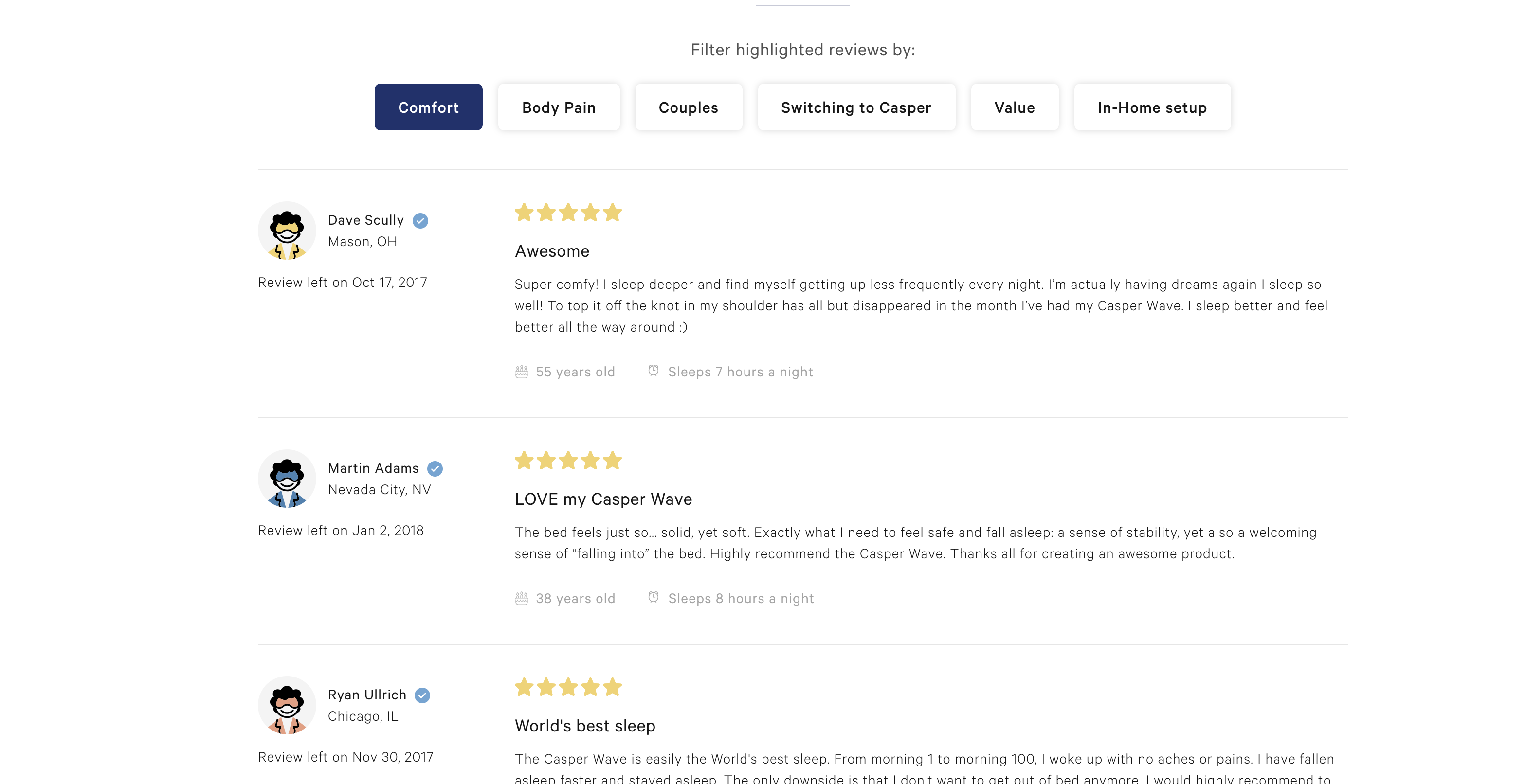Here's a cleaned-up and detailed caption based on the provided information:

---

At the top of the image, a heading reads "Filter Highlighted Reviews by," followed by six filter options: Comfort, Body Pain, Couple, Switch, Switching to Casper, Value, and In Home Setup. The selected filter is Comfort, located on the left side. Below this header, several five-star reviews are displayed, each with yellow stars. 

1. The first review is by Dave Schooley, a verified reviewer from Mason, OH. His review, left on October 17, 2017, is accompanied by an orange and black character icon. He writes:
   "How was Sam? Super comfy. I sleep deeper and find myself getting up less frequently every night. I am actually having dreams again; I sleep so well. To top it off, the knot in my shoulder has all but disappeared in the month I have had my Casper Wave. I sleep better and I feel better all around. 55 years old, sleep 7 hours a night."

2. The second review is by Madzine Adams from Nevada City, NV, left on January 2, 2018. Her icon is blue. She says:
   "Love my Casper Wave. The bed feels just so solid yet soft, exactly what I need to feel safe and fall asleep. A sense of stability yet also welcoming, a sense of falling into the bed. Highly recommend the Casper Wave. Thanks all for creating an awesome product. 38 years old, sleep 8 hours a night."

3. The last review is by Ryan Woolridge from Chicago, IL, left on November 30, 2017. His icon is brown and black. His review reads:
   "World's best sleep. The Casper Wave is easily the world's best sleep. From morning 1 to morning 100, I woke up with no aches or pain. I have fallen asleep faster and stayed asleep. The only downside is that I don't want to get out of bed anymore. I would highly and quickly recommend it too."

---

This detailed caption thoroughly describes the image's layout and contents, providing clear insights into each review and the associated details.